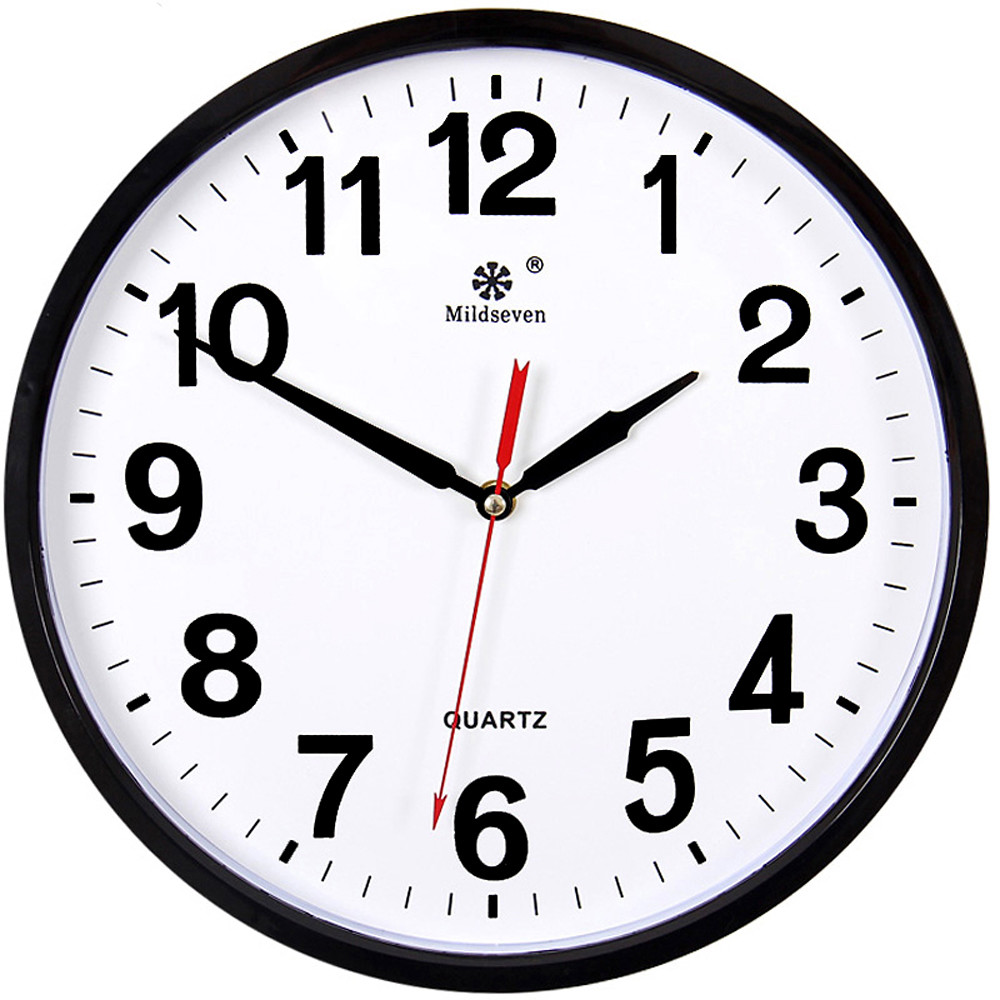This is a detailed description of a round wall clock with a bold black border encircling a white clock face. The clock features bold black numbers and minute notches. The hour hand is a short black hand pointing to the 2, the long black minute hand is near the 10, indicating the time is 2:50, and a slender red second hand is just past the 6. Beneath the 12 at the top, there is a star-like logo followed by the text "Mild Seven." Additionally, just above the 6 at the bottom, the word "Quartz" is displayed.